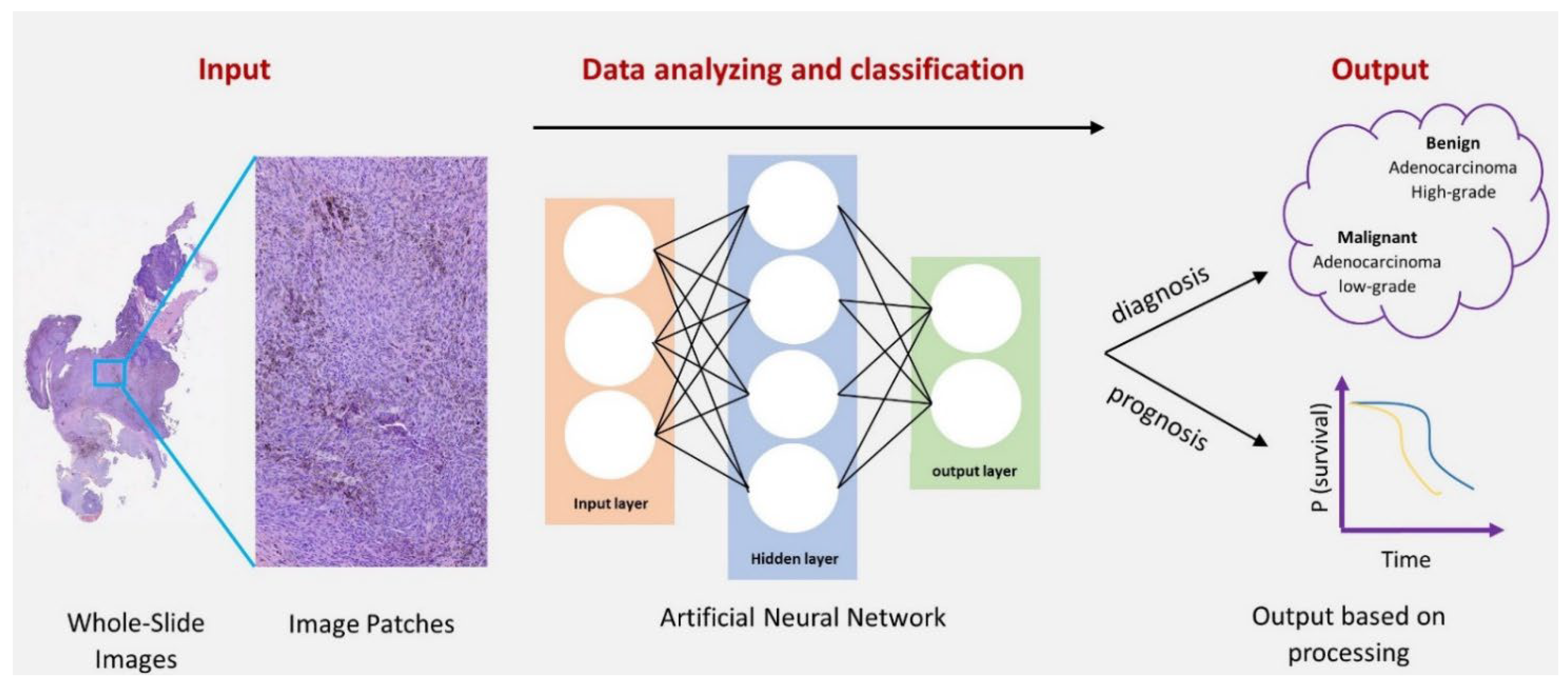The image is a detailed diagram, likely from an academic or scientific context, illustrating the process of medical data analysis and classification, specifically in diagnosing and prognosing cancer. At the top, it reads "Input data analyzing and classification and output." The diagram is divided into three main sections: input, data analysis, and output. 

The input section on the left starts with "whole slide images," depicted as a purple blob, and progresses to more detailed "image patches," represented as a larger rectangular lavender segment. The middle section is dedicated to data analysis, featuring an "artificial neural network" with a series of connected white circles arranged in three layers: input, hidden, and output. This illustrates the complex process of layer-by-layer analysis.

On the right side is the output section, which details "diagnosis" and "prognosis." A cloud-shaped graphic includes diagnostic terms such as "benign adenocarcinoma high grade" and "malignant adenocarcinoma low grade." Below these terms, there's mention of survival rates displayed alongside an L-shaped arrow indicating time at the bottom right corner. This sophisticated diagram dispels how data from whole slide images is analyzed through neural networks to conclude medical outcomes such as cancer diagnosis and survival prognosis.